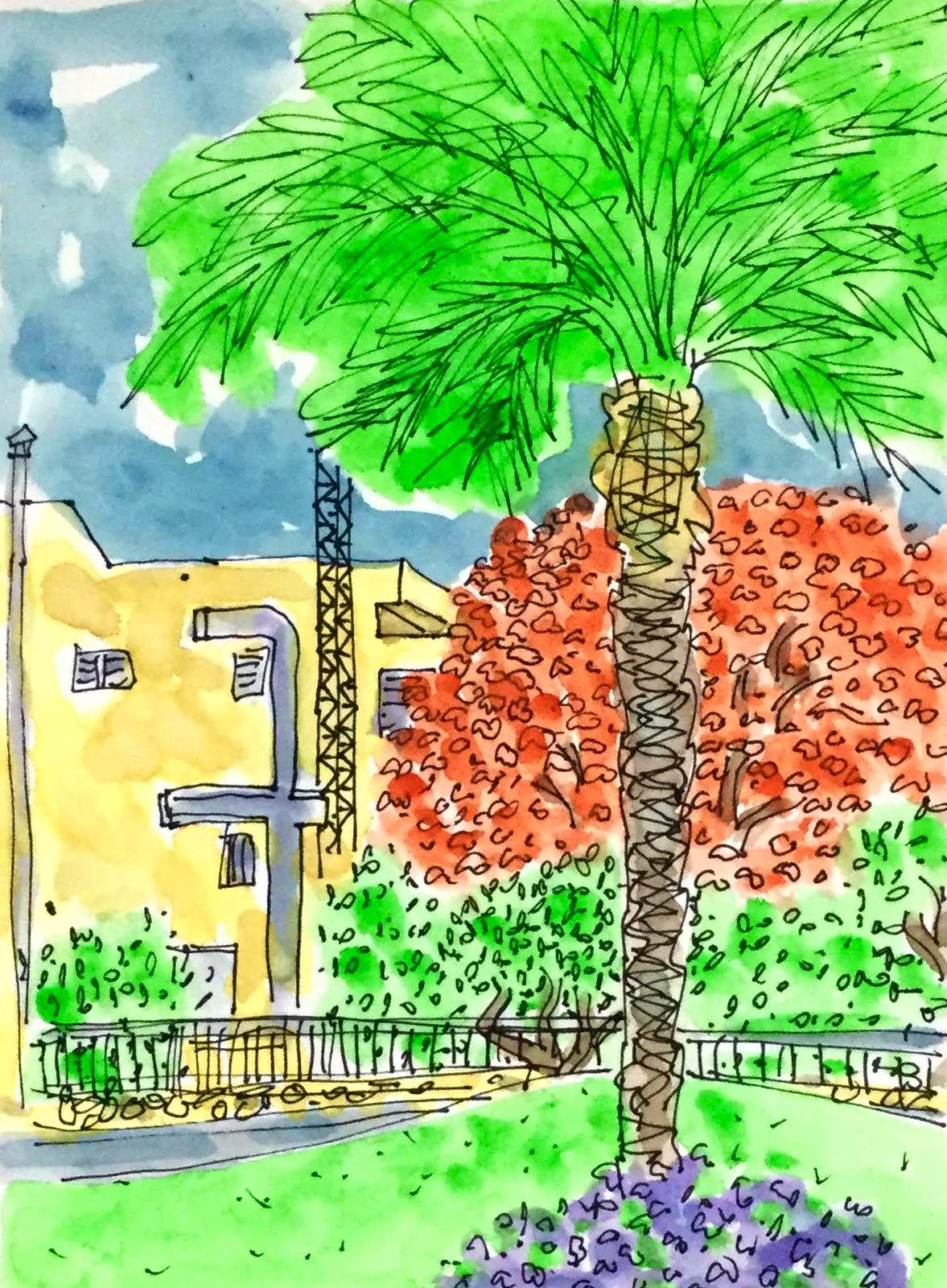A minimalist watercolor painting captures the serene front lawn of an apartment building with striking detail. The building stands prominently with its yellow walls accented by visible metal work, including air ducts and an exhaust system on the side. To the left, a towering red tree adds a burst of color against the structure. A fence delineates the property, and behind it, a graceful palm tree rises on a slight hill. This small elevation appears to be flanked by a walkway or driveway that subtly curves around the tree. Bright blue flowers are nestled near the base of the red tree, adding a touch of delicate beauty. The sky above is rendered in broad, sweeping strokes of blue. The overall composition is defined by basic pencil or pen lines, which guide the viewer's eye, enhanced by the thoughtful addition of color beyond the lines.